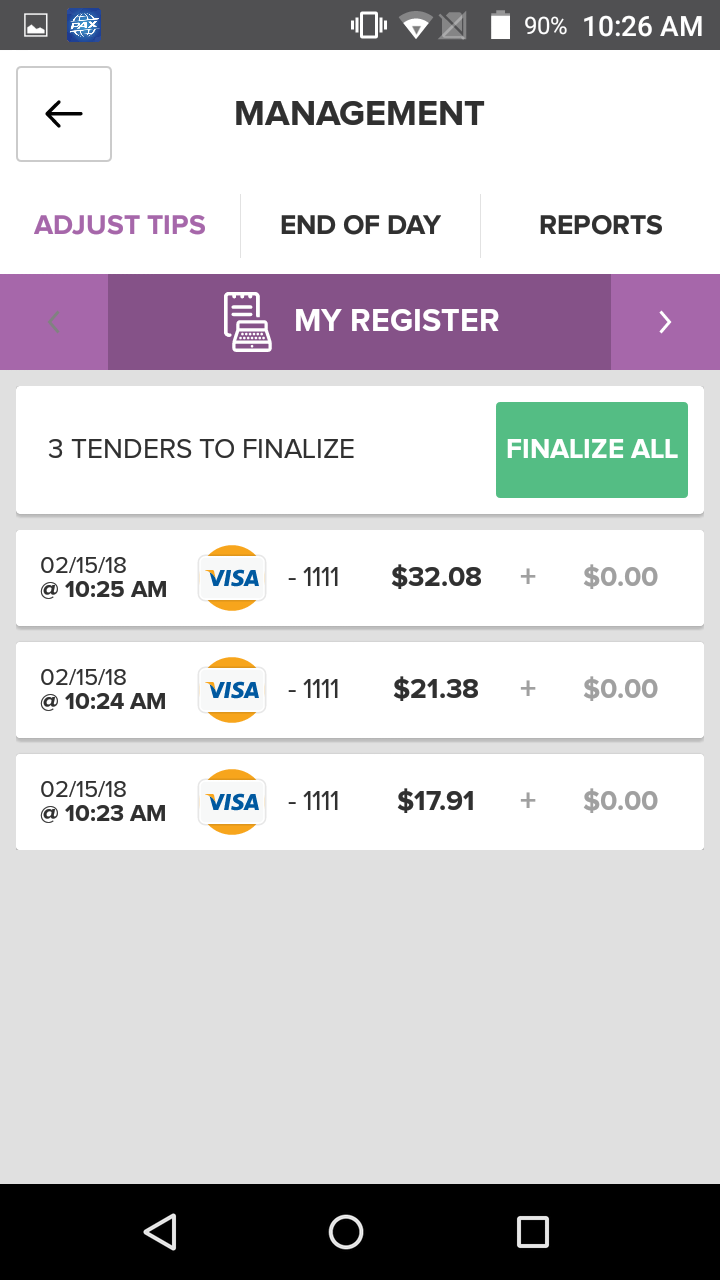This is a descriptive caption for a screenshot from a website, elaborately detailed:

The image is a screenshot capturing a section of a website interface. At the very top, there is a prominent black banner. This banner features a square icon with illustrations resembling houses set against a blue background, accompanied by the text "PAX" in capital letters. Adjacent to this, various status icons can be seen including a Wi-Fi signal, a cell signal with an "X" indicating loss of connection, a vibrating cellphone icon, and a battery indicator showing 90% charge, with the current time displayed as 10:26 a.m.

Moving downwards, there is a square icon containing a leftward arrow. Centrally positioned text reads "Management Capital" in uppercase letters along with "Fold Letters" below it. Further down, the text "Adjust a Day in Reports" is visible, with "Adjust tips" highlighted in purple text while the remaining text is in black uppercase letters.

Proceeding to the next section, a purple banner spans across, prominently displaying "My Register" in the center. Adjacent to this, a smaller purple box with a rightward arrow is apparent. Below this section, the background transitions to gray. On a white banner within this gray backdrop, the message "Three Tenders to Finalize" is visible, alongside a green rectangle button labeled "Finalize All".

Descending further, repeated entries of dates "2-15-18" are listed thrice, each followed by the text "Visa." Below each entry, a series of numbers "3208-21-038-1791" can be seen, signifying what appears to be transaction data.